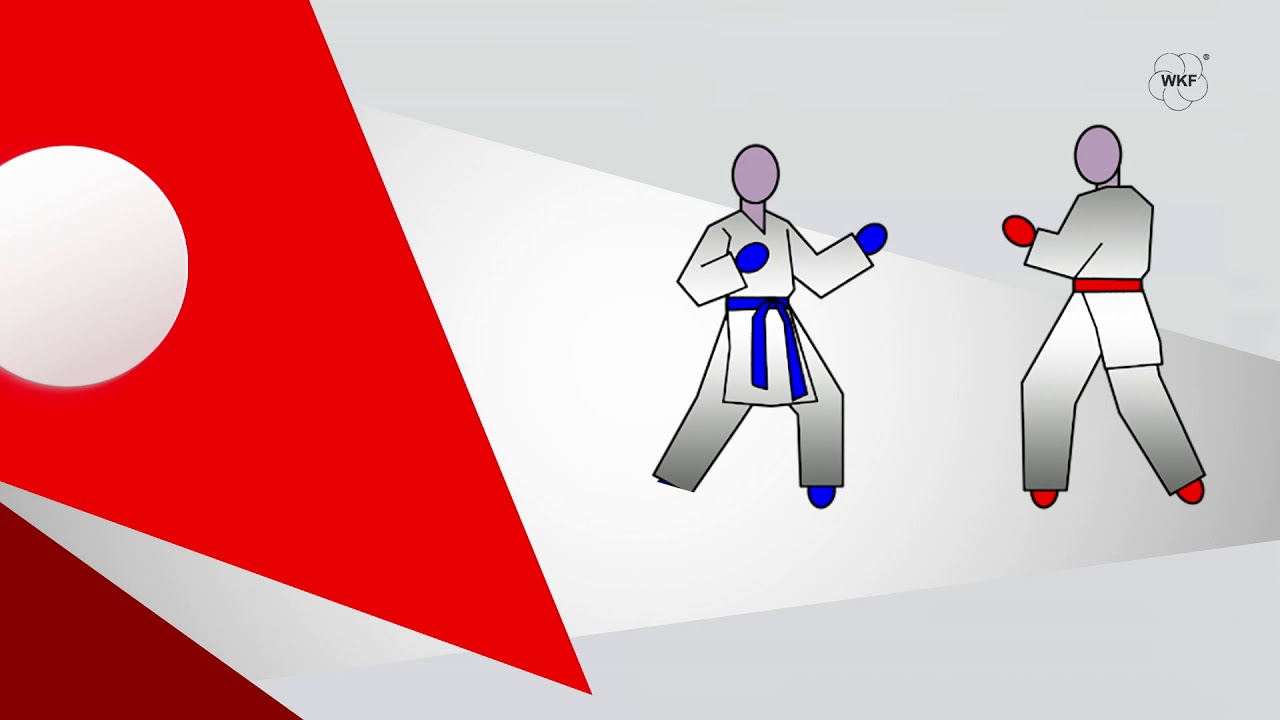The digitally created image features two gender-neutral figures wearing traditional white karate uniforms with long sleeves and pants. They face each other in fighting stances. The figure on the left is distinguished by blue hands, blue feet, and a blue belt, while the figure on the right has red hands, red feet, and a red belt. Both figures have featureless circular heads colored in light pink or light purple. The background is composed of varying geometrical shapes, primarily triangles in shades of grays and whites. On the left side, there are additional red and brown triangular shapes. In the upper right corner of the image, a black logo resembling five petals or circles is accompanied by the text "WKF" in black lettering, enhancing the visual design of the scene. The overall image is bright and clear, making the details easily visible.